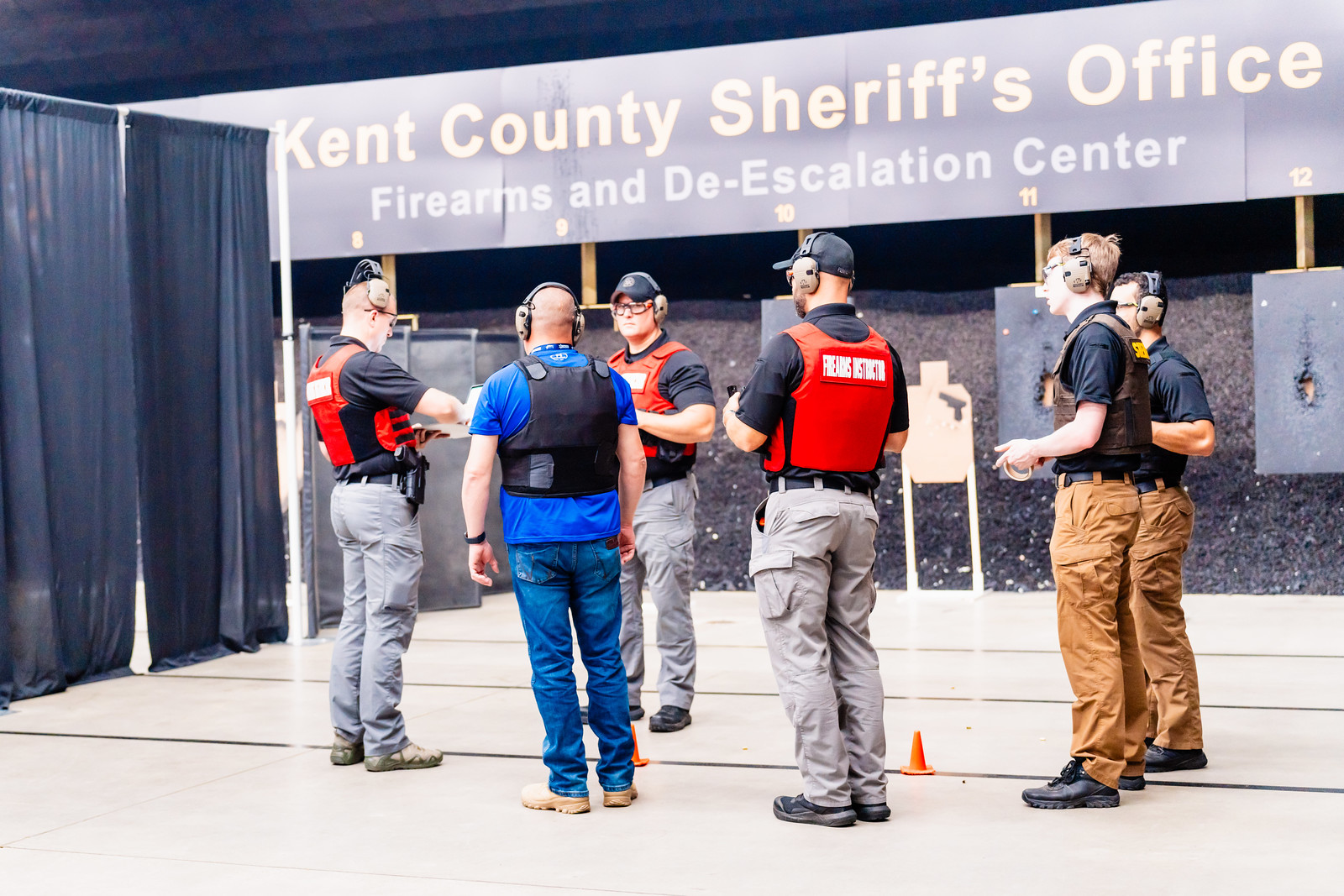This image depicts a group of men standing together at the Kent County Sheriff's Office Firearms and De-escalation Center, as indicated by a sign overhead. The men, who appear to be law enforcement officers in training, are equipped with protective vests and headphones typically used at shooting ranges. The vests vary in color: some are red, some black, and some brown. Underneath these vests, most men are wearing black polo shirts, though one is distinguished by a blue polo shirt. Their pants also vary, with combinations of black, brown, and gray, while the officer in the blue shirt is wearing blue jeans. Many of the men are also wearing safety glasses. Behind them, targets are set up against a backdrop, with a curtain positioned to the side. The group appears to be in a moment of discussion or briefing, rather than actively engaging in firearm practice.